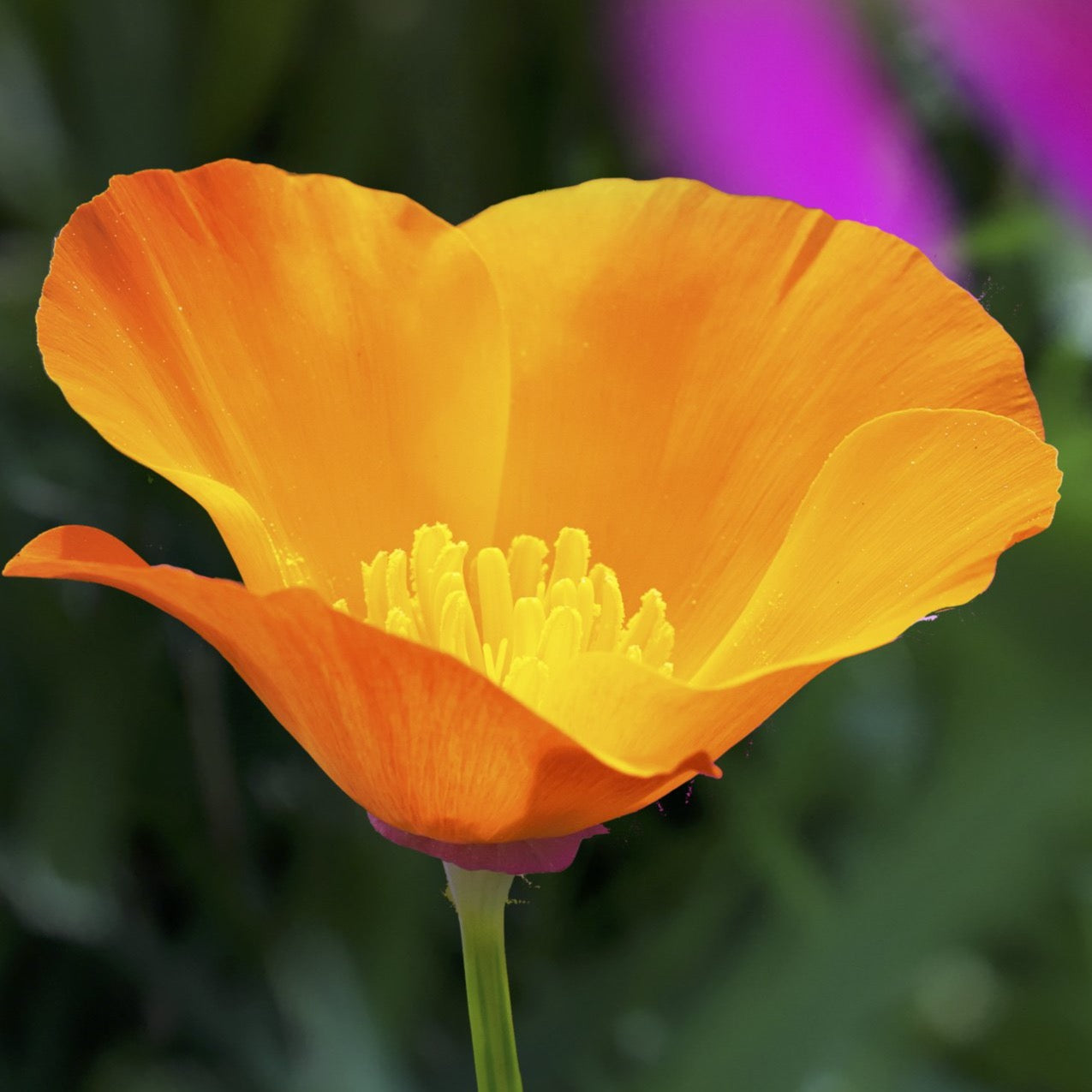In the center of this close-up image, a vibrant orange flower, possibly a poppy, dominates the scene with its delicate beauty. The flower features petals in varying shades of orange, with the darker hues adorning the outer edges and lighter tones gracing the inner areas. The flower has about four large petals arranged in a circular pattern. At the core of the bloom are several yellowish-orange stamens, standing upright like tiny, delicate sticks, hinting at the flower's reproductive parts where pollen is found. Partially visible at the base is a green stem, suggesting that the flower is rooted in its natural setting. The background is intentionally blurred, creating a soft, bokeh effect featuring mostly dark green tones, likely from surrounding grass. Adding a splash of color, a bright fuchsia or violet blur occupies the top right-hand section of the image, possibly from another flower. The left side of the background is darker, almost black, providing a striking contrast that enhances the vividness of the central flower. Overall, the image is a vibrant, detailed depiction of the flower in its natural habitat, captured in the middle of the day.